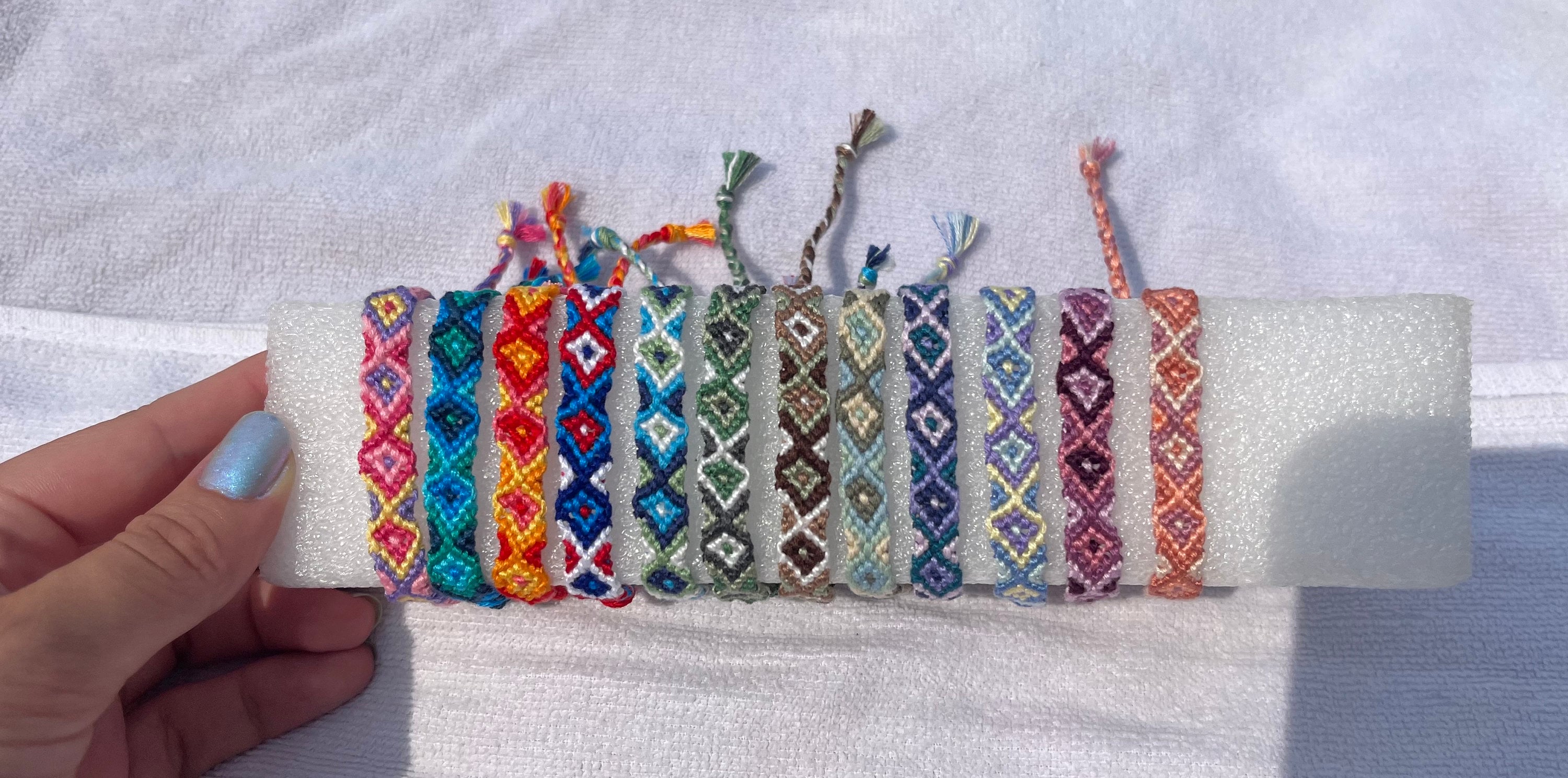The photograph captures an assortment of handmade friendship bracelets displayed on a triangular piece of styrofoam. The bracelets are intricately tied around the styrofoam, arranged from left to right, showcasing a variety of colors and patterns. A woman's hand with blue nail polish on her thumb holds the styrofoam triangle, positioning it against a white, possibly cloth background, likely for an Etsy shop presentation. The first bracelet on the left features beads in pink, red, purple, yellow, and gray with a distinct diamond and arrow pattern. The subsequent bracelets show a range of colors from green to dark green, blues, and aqua, transitioning to an orange bracelet with purple and white designs. The display includes eight more bracelets, each unique in its color scheme, contributing to a vibrant mosaic. Shadows appear on the right side, suggesting possible cropping for a cleaner presentation.